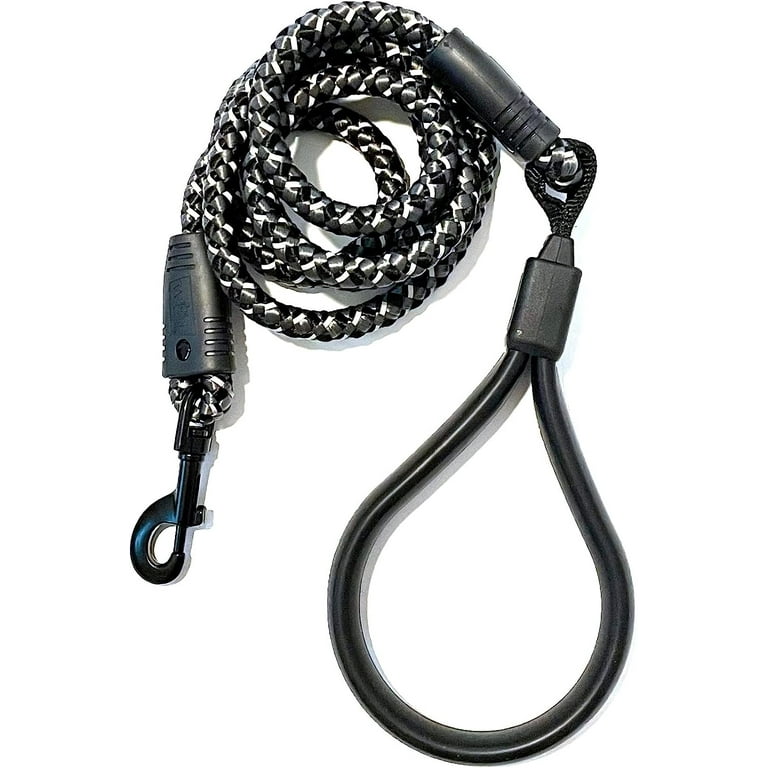The image centrally features a black leather dog leash, prominently displayed against a solid white background. The leash, detailed in the zoomed-in shot, showcases a coiled dark silver chain, which contrasts with the black leather handle forming a large loop. This vertical photograph emphasizes clarity, allowing viewers to inspect the leash's high-quality material and craftsmanship, likely intended for a pet merchandise website. The simple, uncluttered background ensures that the leash is the primary focus, highlighting its potential use and elegant design.